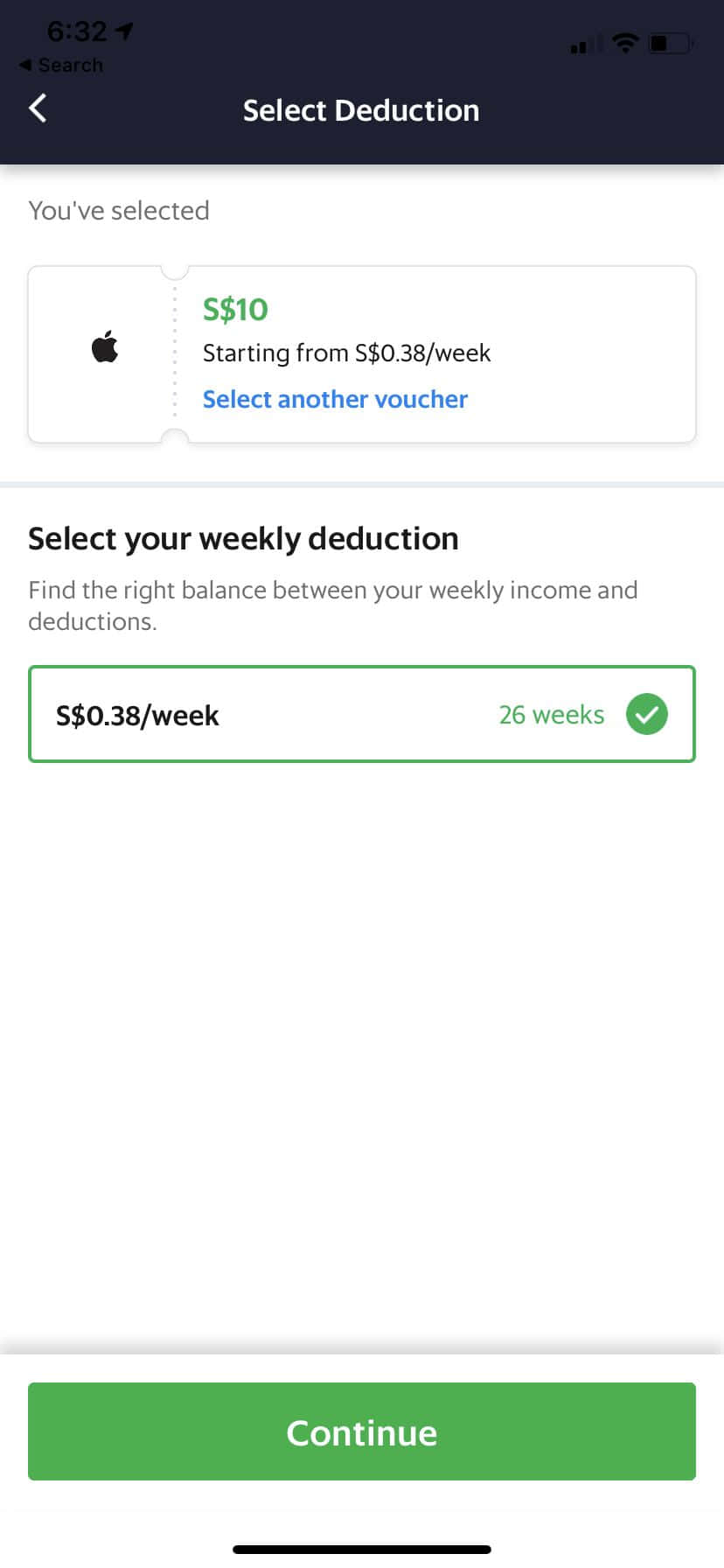This is a screenshot with a clean and detailed user interface. At the top, the status bar displays the time "6:32" in black text, accompanied by a paper airplane icon, WiFi icon, and battery symbol. Below this, a navigation header features a white back button and the title "Select Deduction." The main section informs the user of their selection: a white box with a black Apple logo, labeled "S10" in green text, indicating a price starting from "0.38/week." Beneath this, a blue link invites users to "Select another voucher."

Further down, a black text prompt, "Select your weekly deduction," advises users to balance their weekly income and deductions. This is followed by details in green text: "0.38/week for 26 weeks," accompanied by a green circle with a white check mark, all encased within a green border.

Towards the bottom, a gray divider line separates the form from the action button. A green button labeled "Continue" in white text stands out prominently, with a thin black line below it. The image boasts excellent visual clarity, with no pixelation or blurring, making the text easily readable and highly user-friendly for those with low vision. No additional images or noteworthy elements are present, ensuring the focus remains on the primary content.